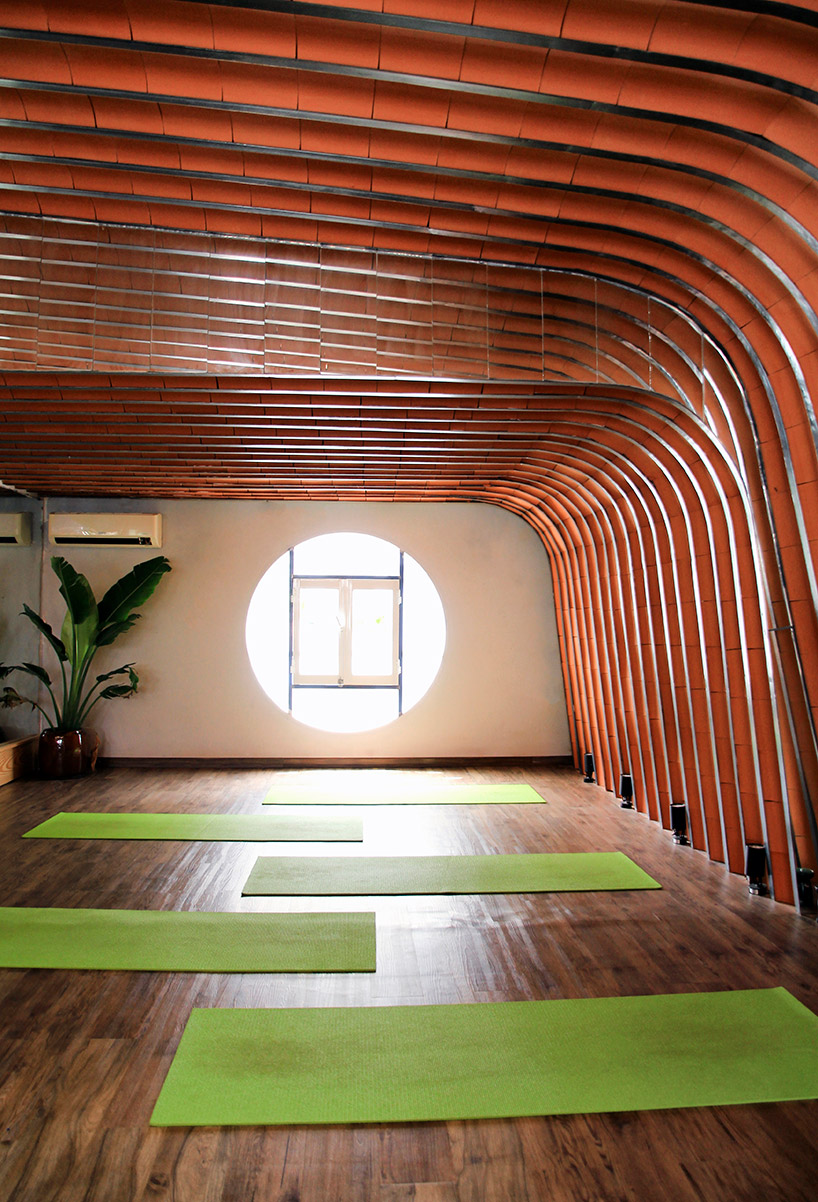This image depicts the serene interior of what appears to be a yoga or prayer studio. The studio features a wooden floor with five forest green yoga mats, each marked by signs of wear with brown patches along the sides and center. In the far corner stands a tall planter containing a large leafy green plant, housed in a brown vase. Above this planter, a white AC unit with a black grate and control panel is affixed to the wall. A large mirror with a wooden base adorns the left side of the studio, reflecting the peaceful ambiance. The beige walls are beautifully accented by a circular window with two square panes, which allow daylight to stream in, indicating it's daytime. The ceiling and walls showcase striking wooden structures that curve downward at the edges, adding both support and aesthetic appeal to the space, creating an overall inviting and healing atmosphere.